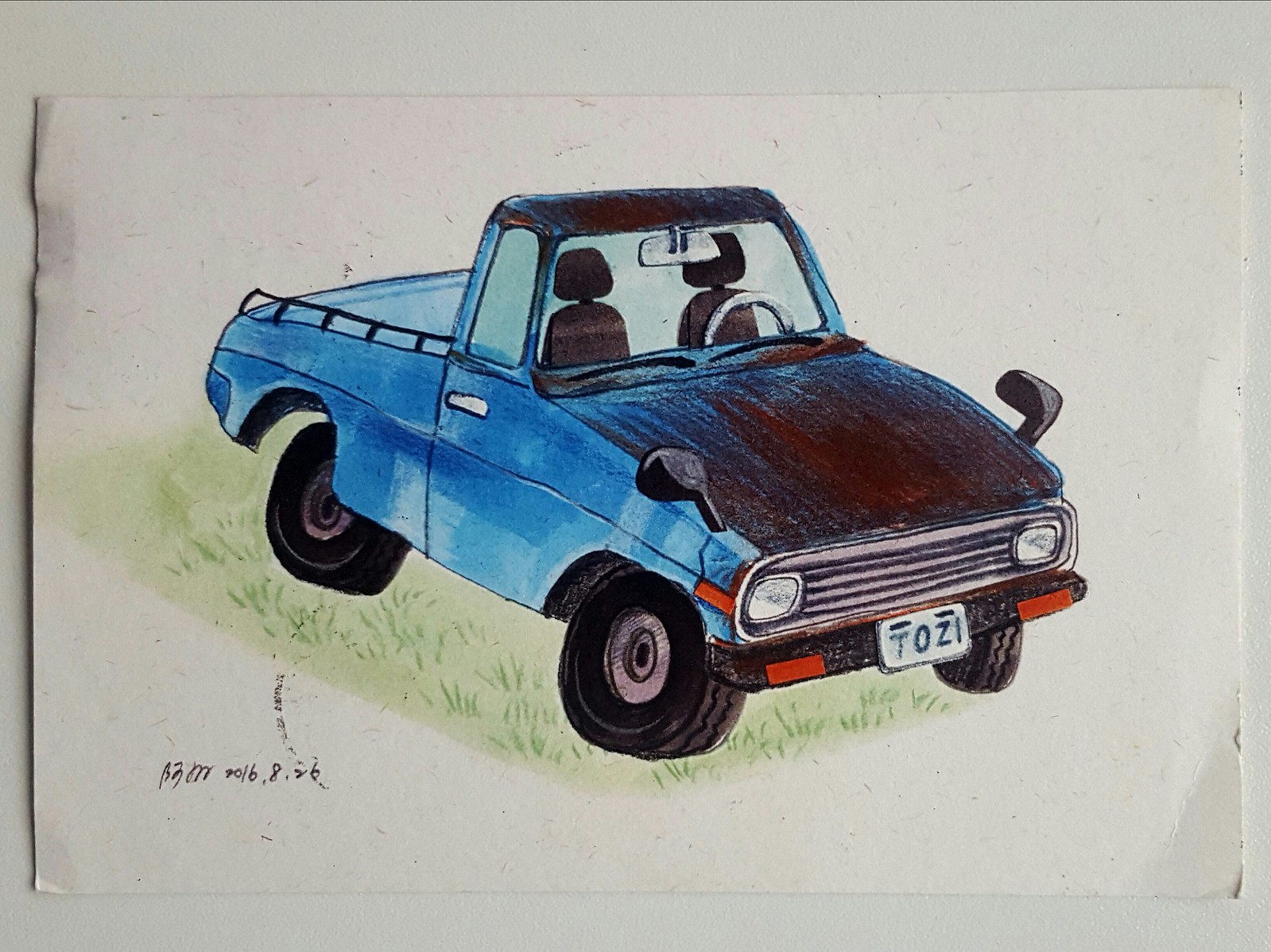This is a photograph of a color drawing of an older type, two-seater utility vehicle, known as a "ute" in Australia, which resembles a small pickup truck or models like older Toyotas or Volkswagens. The truck is blue with a blend of blue and red on the hood and features brown seats and a white steering wheel visible through the windows. The vehicle has four black wheels, though only three are fully visible due to the angle of the drawing. It is adorned with rearview mirrors protruding from the hood on both sides and a black guard rail on the flatbed at the back. In front, there's a black bumper with red reflective strips. The truck is shown parked on green grass. The details include a license plate that reads "TOZI," with lines over the "T" and "Z." The drawing, made with colored pencils and potentially some watercolor paint, is signed by the artist with a date of "2016.8.26."